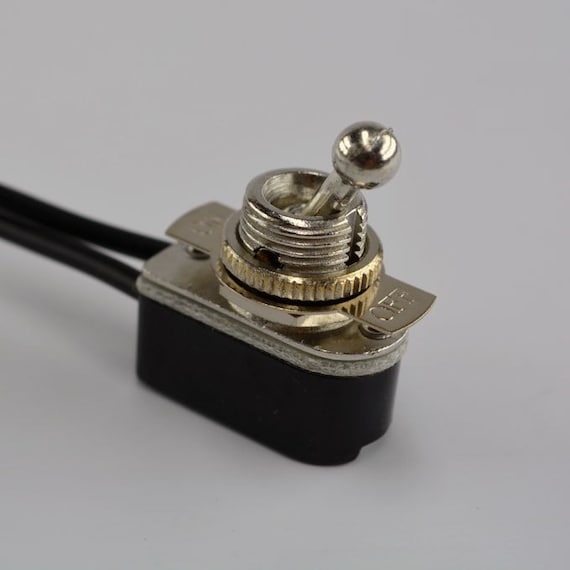This extremely high-quality close-up photograph captures a unique electrical switch or lever, styled somewhat like a joystick. The switch features a shiny, golden ball handle that can be moved up and down, connected to a black plastic base with exposed threading. The base is marked with the engraved words "ON" at the top and "OFF" at the bottom, indicating its function. The entire mechanism appears to be integrated into a black box, from which wires extend, suggesting its use in a circuit or control board—likely not a residential light switch, but more for specialized or industrial use. The object sits on a white surface, highlighted by a light source casting subtle shadows, emphasizing its metallic and plastic components. Notably, the design and construction hint at an antique or precision-engineered piece, adding an air of sophisticated machinery to its appearance.